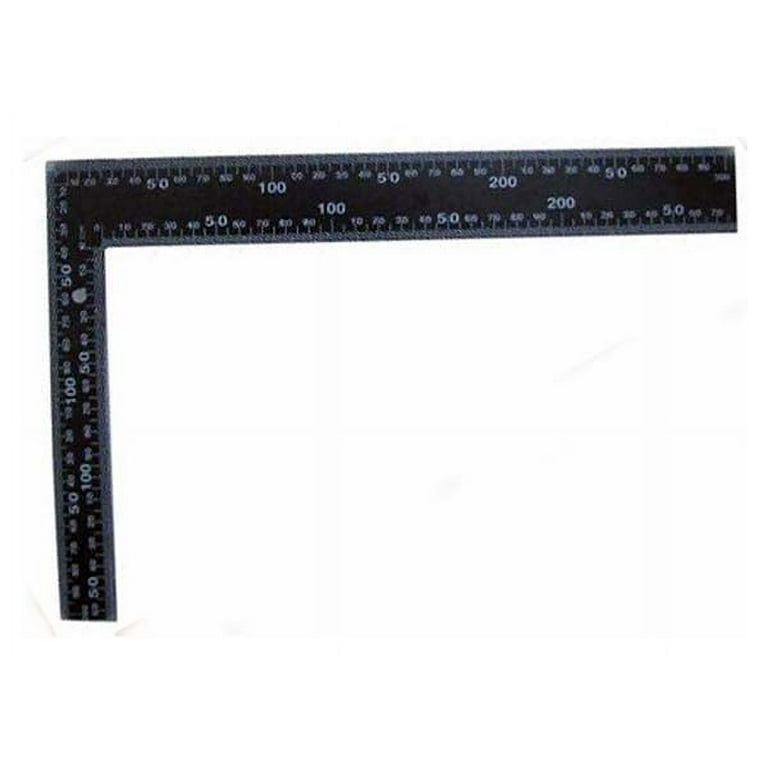The photograph features a black, L-shaped corner ruler, commonly used in carpentry, set against a white, featureless background, creating a stark contrast. The ruler, extending from the upper left corner both horizontally and vertically, is marked with white measurements in millimeters. The longest side reaches up to 300 millimeters, while the other side extends to 200 millimeters. Both sides display numbers prominently in increments of 50, with especially bold markings at each 100-millimeter point, distinguishing the measurements clearly.